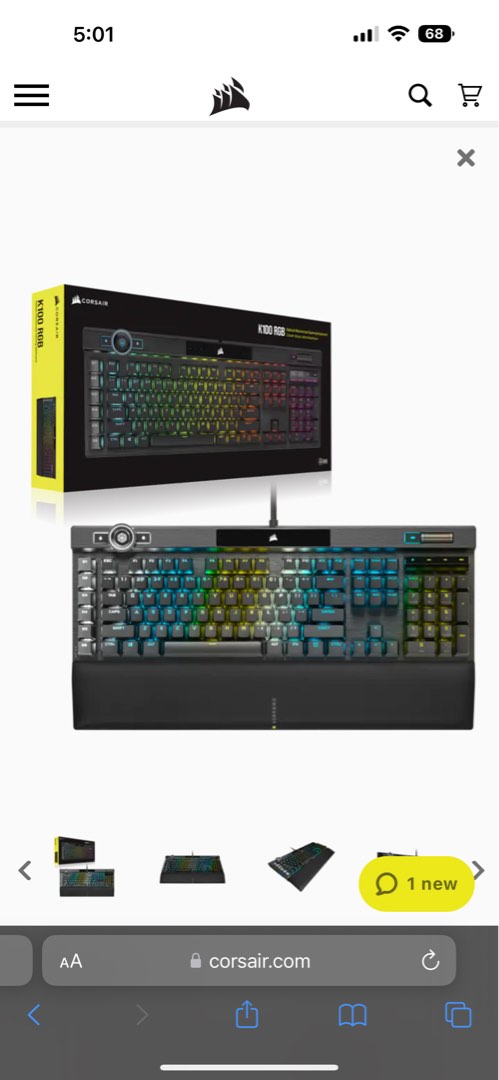**Detailed Caption:**

The screenshot, taken from a smartphone, predominantly features a white background and showcases two primary images centered on the screen. The first image depicts a backlit keyboard, model number K100 RGB, housed in its retail packaging. The box's front face is black and prominently displays a vibrant color image of the gray keyboard with its keys brilliantly illuminated. The side of the box is a striking bright yellow, and the brand name, "Corsair," is clearly visible. The Corsair logo also appears at the top of this smart page.

Directly beneath the box image, there is a top-down view of the actual keyboard. The keys are lit up in a stunning rainbow pattern, featuring hues of blue, yellow, and white. The keyboard is equipped with a palm rest, distinguished by a prominent vertical white line running down its center.

Further down, below the main images, there are four smaller selectable images, each providing additional views or features of the product. At the bottom of the screen, there is a gray search button labeled "Corsair.com." Finally, the navigation bar for the phone is visible at the very bottom of the screen, showcasing forward and reverse arrows, page up functions, and other navigation tools.